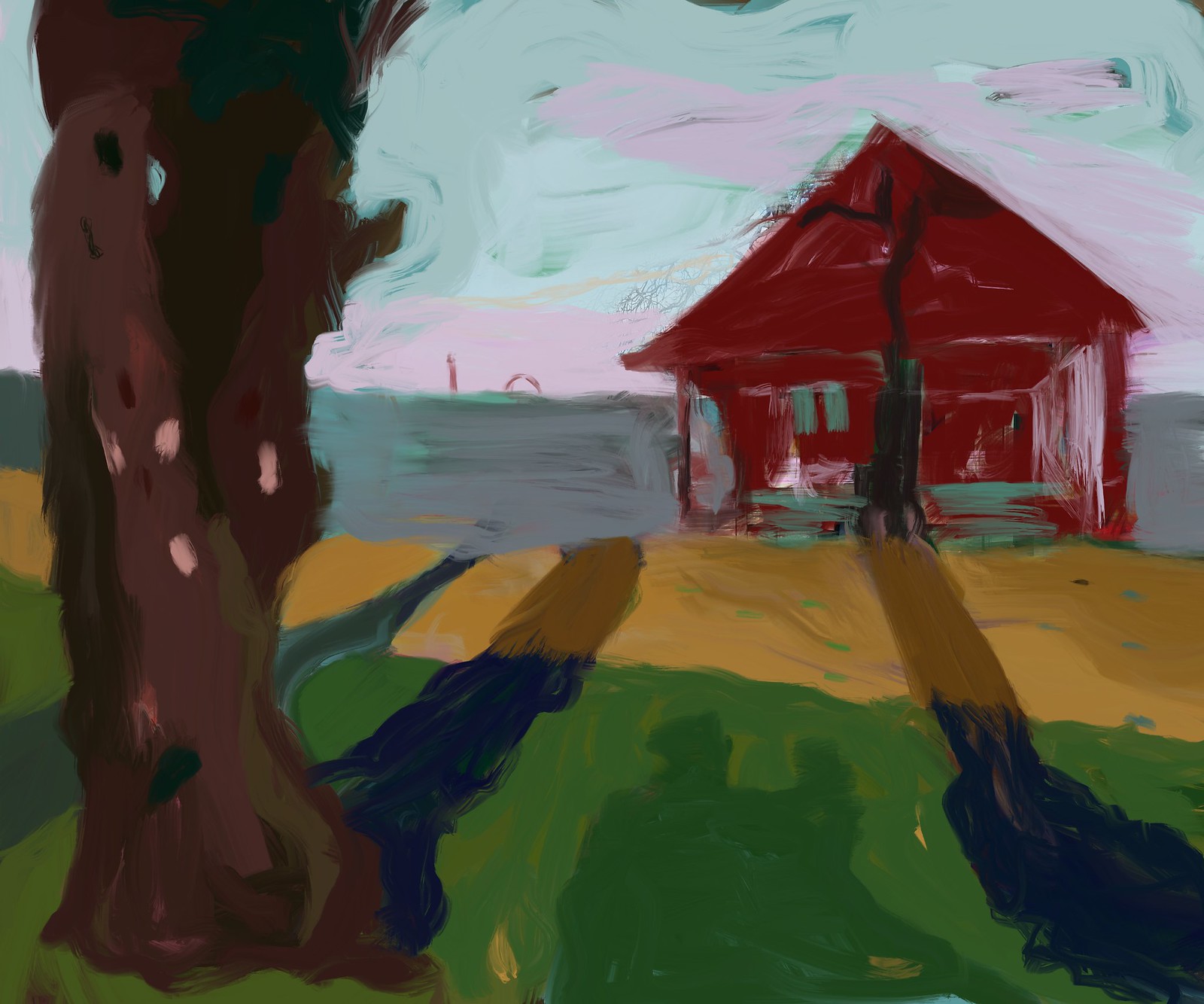The image appears to be a vibrant child's drawing, skillfully painted or colored. The sky is a radiant mix of blue with hints of pink, transitioning into a serene water scene in the background. Dominating the scene is a large brown tree adorned with an eclectic mix of green, blue, brown, and pink hues, giving it a whimsical charm. 

In the foreground, tiny figures or objects in green, blue, and brown can be seen energetically scattered across a yard filled with green grass. This yard stretches up to a quaint red house characterized by its green windows and a small green splash across the front. The house also features patches of white paint on one wall and a slender tree growing along its facade. The area in front of the house alternates between patches of brown and green grass, with a prominent shadow casting across the scene, adding depth and intrigue to the drawing.